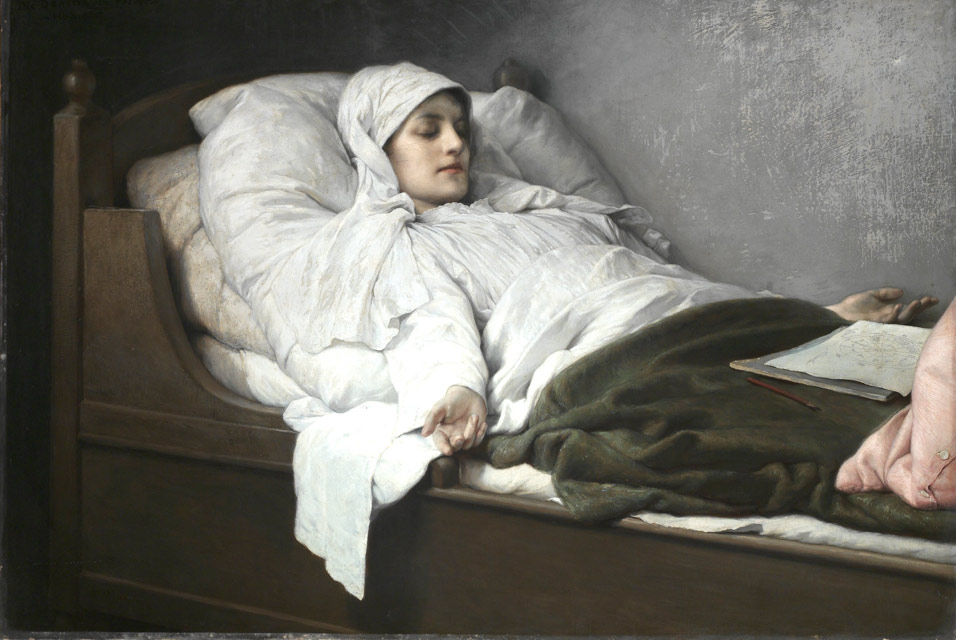This highly detailed and lifelike painting depicts a serene woman lying in an old-style wooden bed. She is dressed in a white, long-sleeved nightgown with a white shroud draped over her head, giving her an ethereal, almost religious appearance. The woman is propped up on two or three large pillows, with her eyes peacefully closed and her arms outstretched, palms up, suggesting she might be either in a deep sleep or unwell. Her dull red lips and fine Roman nose hint at her quiet beauty.

The bed is adorned with a brown bedspread, pulled up to her waist, and a green, fuzzy blanket laid over it. Above her knees rests a pink pillow, adding a subtle splash of color to the scene. On her lap, atop the green blanket, lies a notebook with papers and a pencil or paintbrush, indicating she was sketching or making notes before reclining.

The setting appears to be within a room with gray and bleach-white walls, possibly suggesting an old Italian, French, or medieval village. The wall behind the bed is dark and indistinct, adding to the timeless, historical feel of the image. This evocative scene, reminiscent of a 17th-century portrait, leaves viewers pondering whether the woman is merely sleeping or in a state of repose due to illness, making it a deeply intriguing and poignant composition.